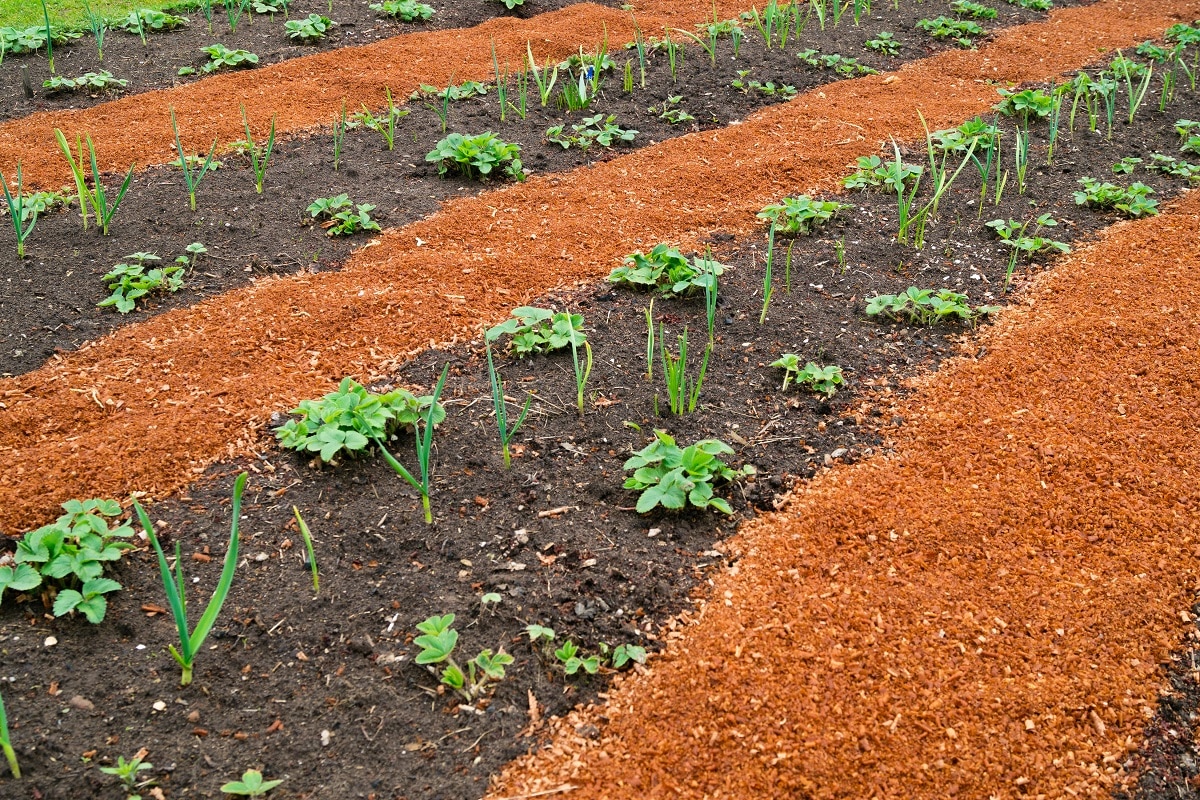The photograph captures a meticulously maintained and organized daytime view of a farmland field, showcasing multiple neat rows of alternating colors and textures. Starting from the top left corner, the field alternates between strips of green grass and various shades of brown dirt and mulch. The rows of brown dirt feature neatly planted green crops, including what appear to be green onion and cilantro or basil. Each basil plant boasts about 20 or 30 leaves, while the green onions display robust, supermarket-like stems. The alternating pattern of greenery and earthy tones repeats across the field, highlighting the early growth stages and careful organization of this well-tended patch of farmland.